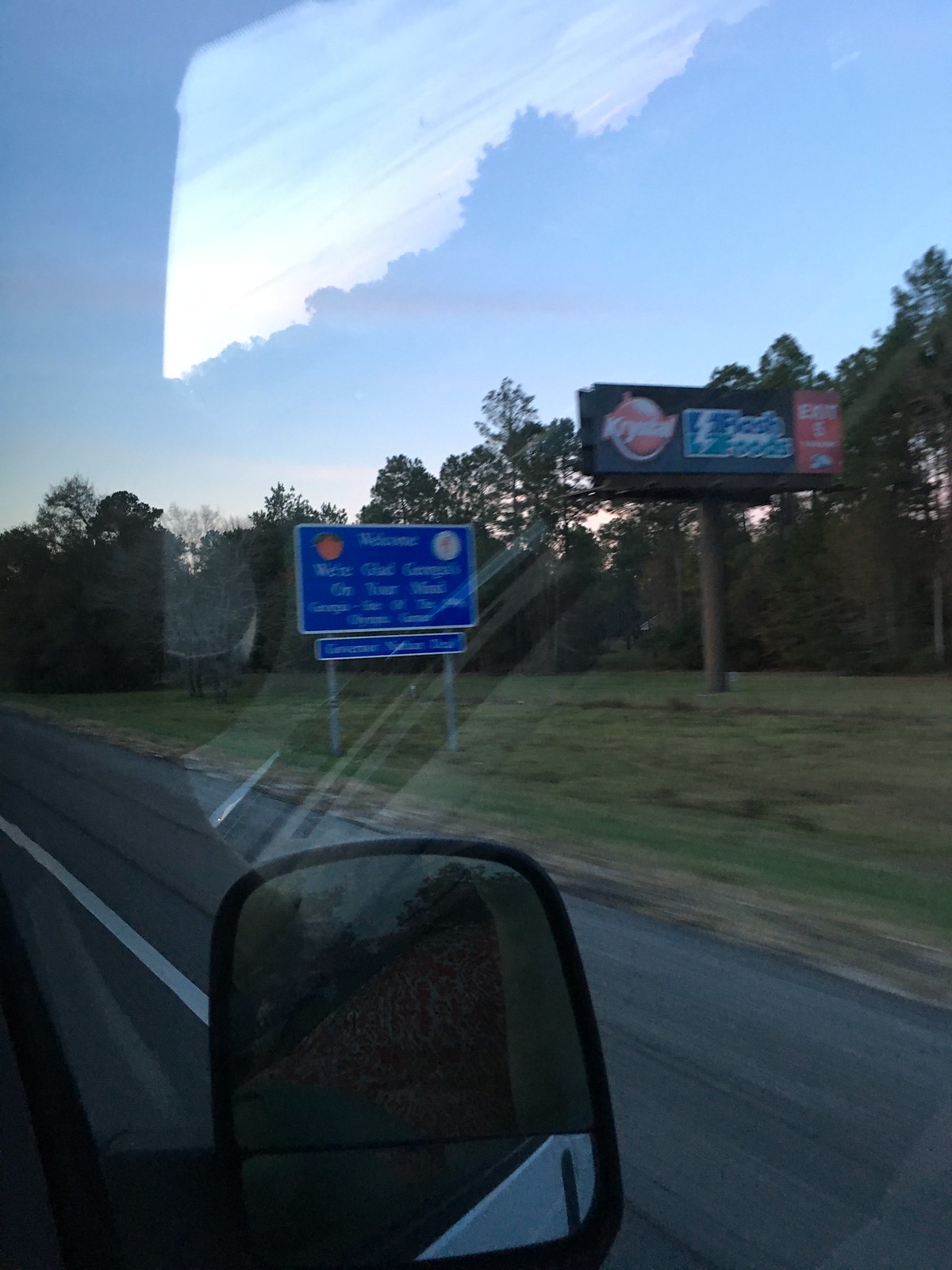Captured from the passenger seat of a vehicle, this image shows the view through a closed window, as evidenced by the reflections on the glass. The car is traveling along a roadside, with part of the passenger side mirror visible at the bottom left of the frame. Prominently featured near the edge of the road is a bright blue welcome sign, signaling the entry into a new area. To the right of the welcome sign stands a large billboard, adding to the roadside attractions captured in this still. The overall scene beautifully encapsulates a typical drive, highlighting the roadside markers that guide travelers on their journey.